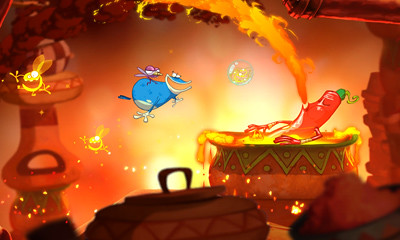The image is a colorful and dynamic digital artwork, likely a screen capture from an animated movie or video game. Central to the composition is a cauldron situated on the right half of the frame, containing an animated red chili pepper adorned with a green hat, exhibiting vivid personality with arms and a face. The chili pepper is immersed in molten lava, dramatically spewing flames from its mouth, which transform into billowing dark smoke clouds in the upper left corner. Accompanying this fiery spectacle is a vibrant scene filled with animated characters. To the left, a vertical vase-type pottery stands out, with a small yellow firefly-like animation hovering in front of it. Scattered across the scene are two more similar firefly animations, one intriguingly trapped inside a soap-like bubble. Adding to the lively atmosphere is a blue bird-like creature flying towards the chili pepper. The background, taking up most of the frame, suggests they are inside a volcano, indicated by structural details reminiscent of volcanic landscapes. The overall scene, though whimsical and fantastical, is meticulously detailed, creating an engaging visual narrative.